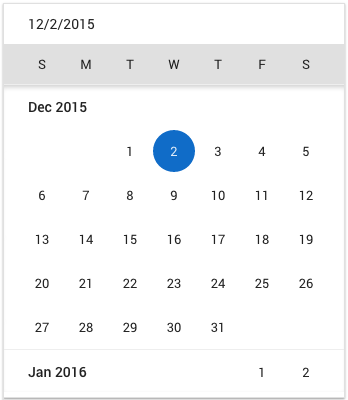The image features a calendar for December 2015, presented in a vertically-oriented rectangular box slightly larger than a square. At the top of the calendar, "12-2015" is displayed. Directly beneath this, there is a purple bar containing the initials of the days of the week: "S M T W T F S." Below the purple bar is the title "December 2015."

The layout shows that December 1st falls on a Tuesday and December 31st falls on a Thursday. Notably, the 2nd of December is highlighted with a prominent blue circle, indicating it is a Wednesday.

At the bottom of the calendar, there is a brief preview of the following month, January 2016. This preview reveals that January 1st falls on a Friday and January 2nd on a Saturday.